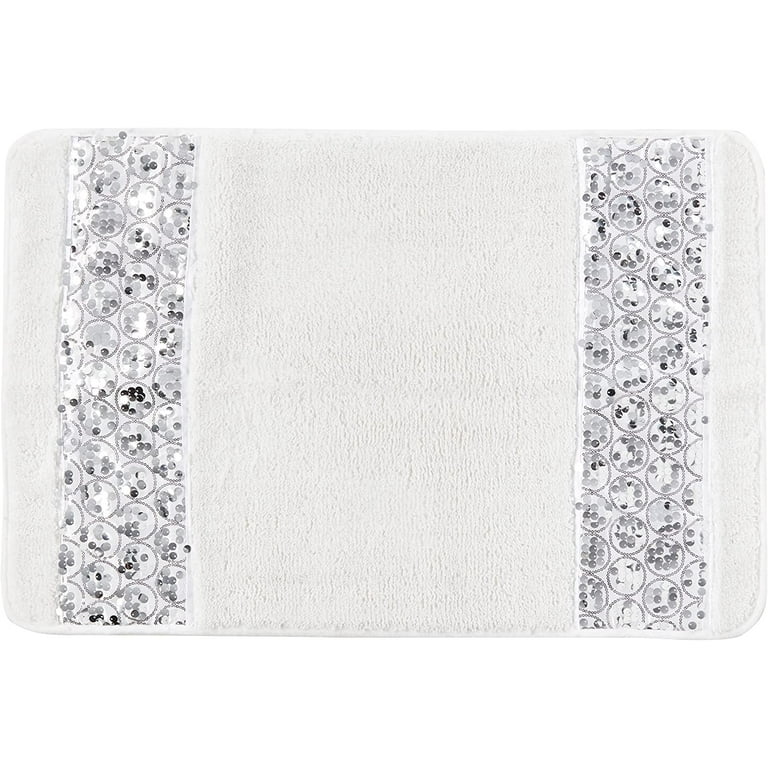This is a detailed image of a white, rectangular mat with slightly curved corners, possibly intended for use as a placemat, floor mat, or bathroom mat. The mat features two thick, vertically oriented strips on its left and right sides, running from top to bottom. These strips are decorated with intricate patterns consisting of four vertical rows of circles. Inside each of the larger circles are smaller circles or additional decorative elements. These internal patterns are adorned with small, shiny items in varying shades of black and gray. The mat has a plush, soft texture, adding to its aesthetic and functional appeal.